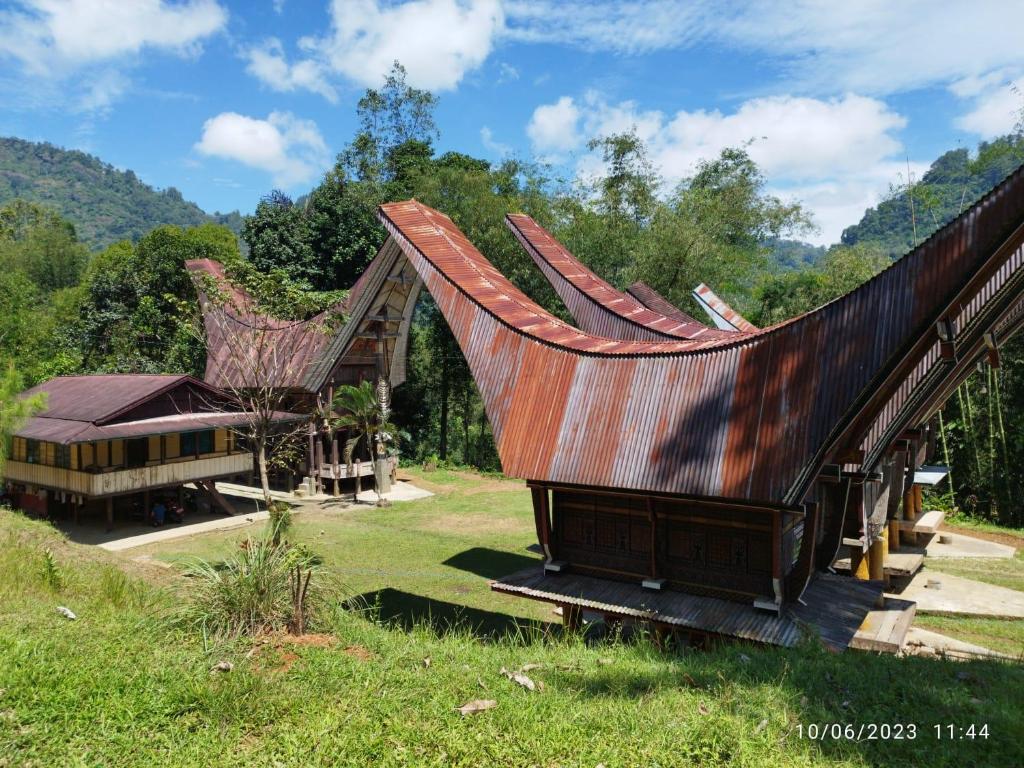The photograph, taken on 10.06.2023 at 11:44 AM, captures a scene of unique architectural structures set in a heavily forested, rural area. The camera is positioned on a grassy hill, looking down onto a small valley where the buildings are nestled. The sky above is a vibrant blue with scattered puffy clouds, suggesting a sunny summer day.

In the center, there are two sets of buildings creating an alleyway between them. On the right, four long, rectangular, two-story buildings stand out with their unusual roof shapes, resembling giant saddles or skateboard ramps. These roofs, made of what appears to be rusted corrugated tin, feature severe angles and a scalloped shape, with streaks of gray and rust-red coloring, likely from oxidation. The bases of these structures are wooden, though details are obscured by shadow.

To the left, there is a more traditional-style house, raised off the ground on short stilts. This house has a yellow, railed-in porch with ample windows and a red shingled, triangular roof, exuding a quaint beach house charm.

Together, these structures blend rustic wooden textures with the striking, weathered metal roofs, all framed by the surrounding trees and small wooded hills, giving the scene a feeling of remoteness and tranquility.